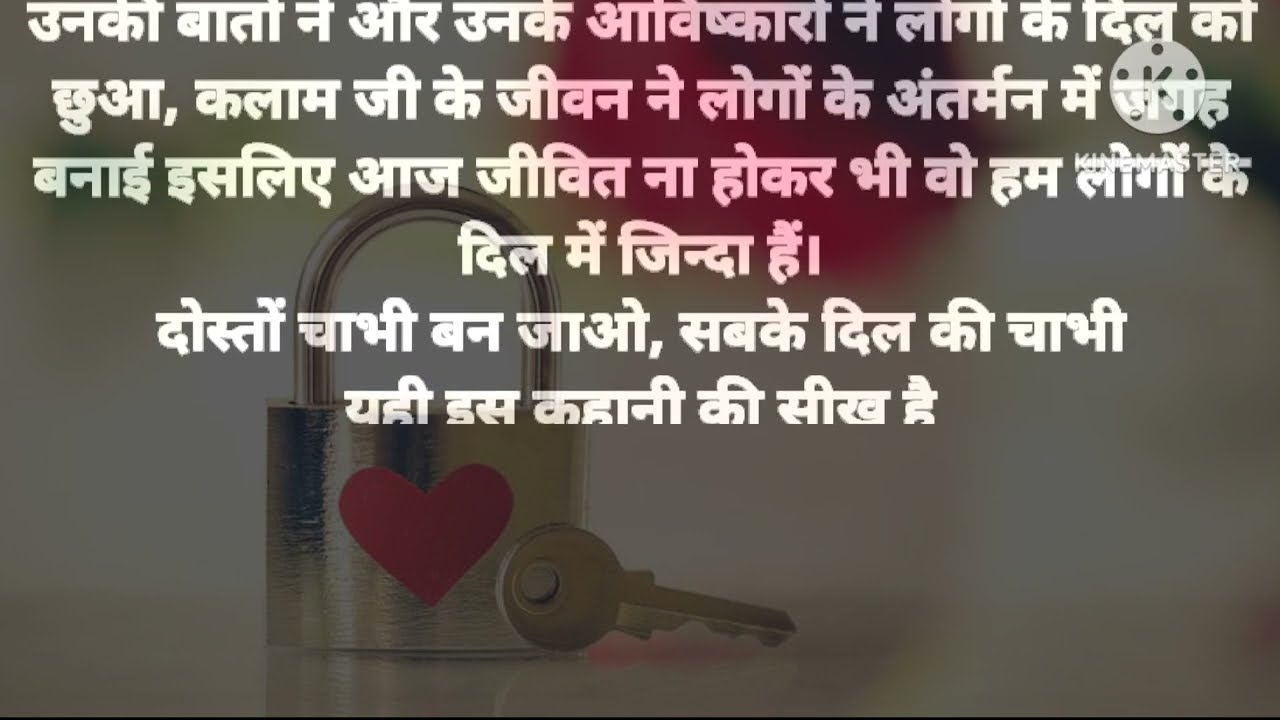The image features a grayish background, with a surface resembling a countertop, though it's mostly blurry and indistinct. In the bottom left corner, there is a gold padlock with a large red heart painted on its front. Leaning against the padlock is a matching gold key. The overall composition suggests that the objects are placed on a smooth surface, like a desk or table. Dominating the top portion of the horizontal rectangular image are six centered lines of white text in an unfamiliar language, characterized by straight lines and occasional commas. The background also contains abstract shapes, with notable red and green tones, further blurred and adding to the overall indistinct and fuzzy appearance. The image's style hints at an inspirational message, possibly intended for sharing on social media.